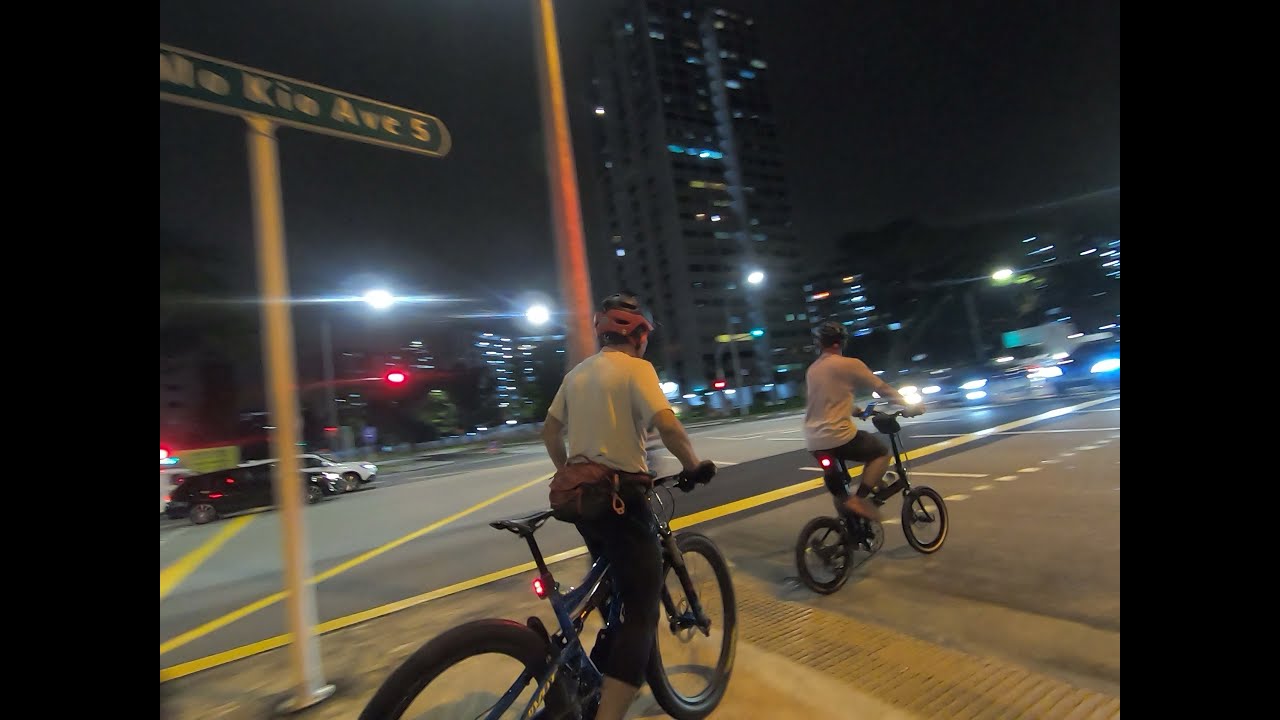The image is a wide, rectangular nighttime photograph of two people riding their bikes in a city. The photo is framed by tall black rectangles on the left and right sides. The road they are riding on starts at the bottom left corner and extends towards the center-right of the image, bordered by a checkered white line, suggesting it might be a designated bike lane or path. A green street sign with white font is visible on the left side, though the text is unclear. On the opposite side of the road, there is a highway with cars moving in both directions, and in the distance, a tall gray building with some illuminated windows dominates the backdrop. Other small buildings and stop lights are also present, creating a bustling urban atmosphere. Both riders are dressed in white shirts and either black pants or shorts, and they are wearing helmets. One rider, also carrying a fanny pack at the back, is off the bike, possibly walking or paused, while the other is riding a small-wheeled trick bike. The scene is set with city lights and a sense of activity, capturing a typical urban night.